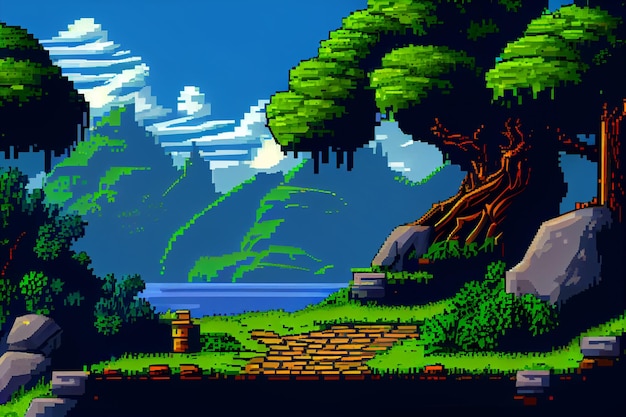The image depicts an old-style, likely 16-bit video game animation of a scenic forest. The scene is pixelated, characteristic of classic video game graphics, with a richly detailed background. At the bottom of the screen, a small golden brick pathway extends halfway through a grassy field. Prominently, the right side showcases a large, majestic tree with a robust trunk and three layers of foliage. Beneath it and to the side are two stones, partially concealed by shrubs. The left side features the overhang of another tree, with some of its branches and a sizable bush visible, and a few stones scattered towards the bottom left corner. The backdrop includes a serene body of water, likely a lake, framed by tall, green mountains. The sky above is a vivid blue, adorned with white clouds, enhancing the tranquil atmosphere of the scene.